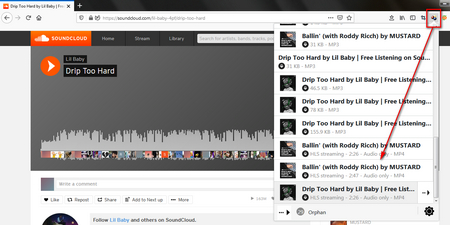The image displays a screenshot from the SoundCloud app. At the top, there is an orange square bearing the SoundCloud logo, while a black navigation bar reads "Home," "Stream," and "Library." Below the navigation bar, there is a track titled "Drip Too Hard" by Lil Baby, with options to repost, share, or add to "Next Up." The interface also includes thumbnail images of individual tracks, featuring artwork with grassy or pointy textures. 

On the top right, a red square encloses additional controls, and the image is bordered visibly. A highlighted section showcases "Ballin" featuring Roddy Ricch by Mustard. The track "Drip Too Hard" by Lil Baby is mentioned repeatedly, emphasizing its availability for free listening on SoundCloud. Additionally, a scroll bar is positioned on the right, and aligned with a red arrow indicating the image's scrolling capability.

Overall, the screenshot encapsulates the SoundCloud user interface, focusing on the availability and features surrounding the tracks "Drip Too Hard" by Lil Baby and "Ballin" featuring Roddy Ricch.